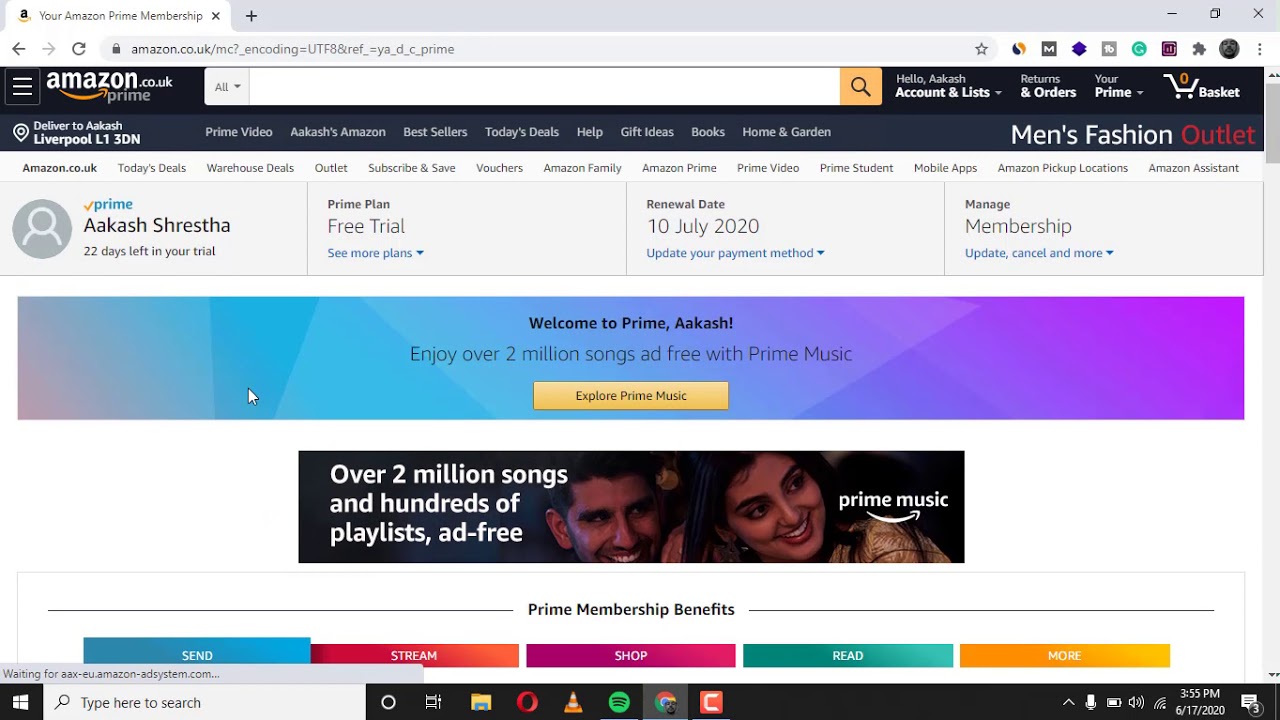The image depicts the Amazon.co.uk website with specific elements highlighted. In the upper left corner, there is a black area displaying the Amazon logo and a Prime label. Adjacent to this is a white search bar featuring an orange magnifying glass icon. The navigation bar includes options such as "Hello Akash, Account & Lists," "Returns & Orders," "Your Prime," and a basket icon showing a quantity of zero. A delivery notification bar states, "Delivered to Akash, Liverpool, L1 3DN."

Below this, a horizontal menu displays various sections of the site, including Prime Video, Akash's Amazon, Best Sellers, Today's Deals, Help, Gift Ideas, Books, and Home & Garden. A "Men's Fashion Outlet" banner is also visible in the top right corner.

Further down, an area indicates Prime membership details for Akash Shrestha—specifically, 22 days remaining in the free trial, with a renewal date of July 10, 2020, and a prompt to manage membership. A welcome message highlights Prime Music benefits, including access to over 2 million ad-free songs and hundreds of playlists. An advertisement featuring a man and woman looking to the right emphasizes these music features.

Beneath this, benefits of Prime membership are summarized with icons and titles for Send, Stream, Shop, Read, and More. At the very bottom, the image captures the toolbar of a computer screen, displaying various system icons.